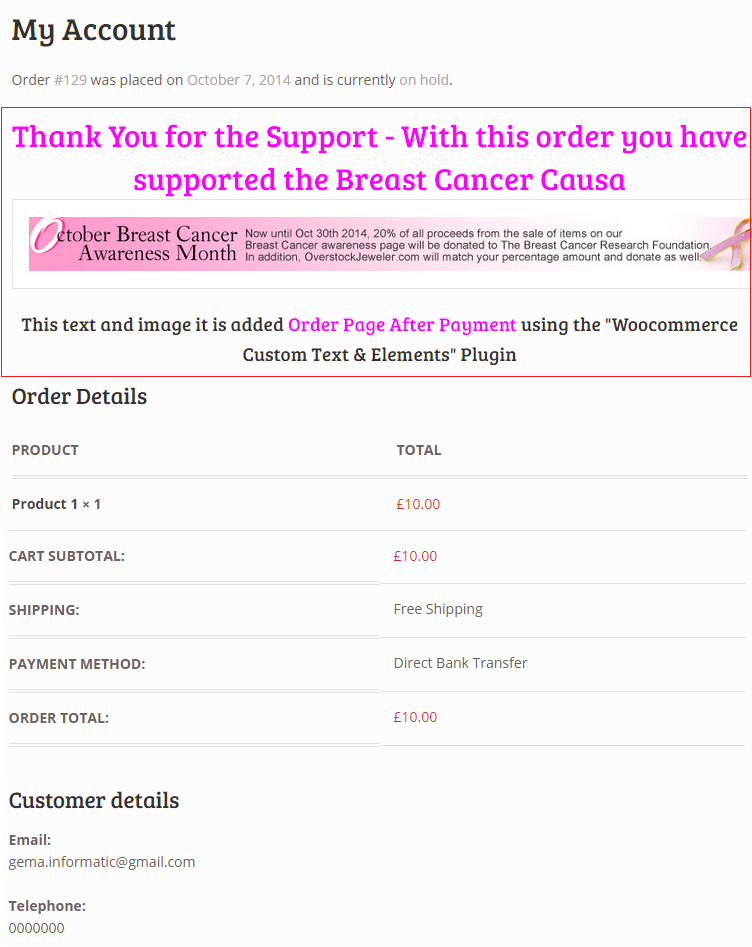Here is a detailed and cleaned-up caption for the given image:

"A screenshot of a web page labeled 'My Account' is displayed on a computer screen. At the top, it indicates that order number 129 was placed on October 7th, 2014, and is currently on hold. Below this, a red box is followed by a message in pinkish text, which reads, 'Thank you for the support - with this order you have supported the breast cancer causa,' highlighting an apparent typo where 'causa' is used instead of 'cause.' The message continues, 'It's October breast cancer awareness month. Now until October 30th, 2014, 20% of all proceeds from the sale of items on our breast cancer awareness page will be donated to the Breast Cancer Research Foundation. In addition, overstock.jeweler.com will match your percentage amount and donate as well.' Further down the page, the order details are displayed, listing a product quantity of one at a price of 10 pounds. The cart subtotal reads 10 pounds, with free shipping noted in the shipping area. Finally, the payment methods section shows an order total of 10 pounds."